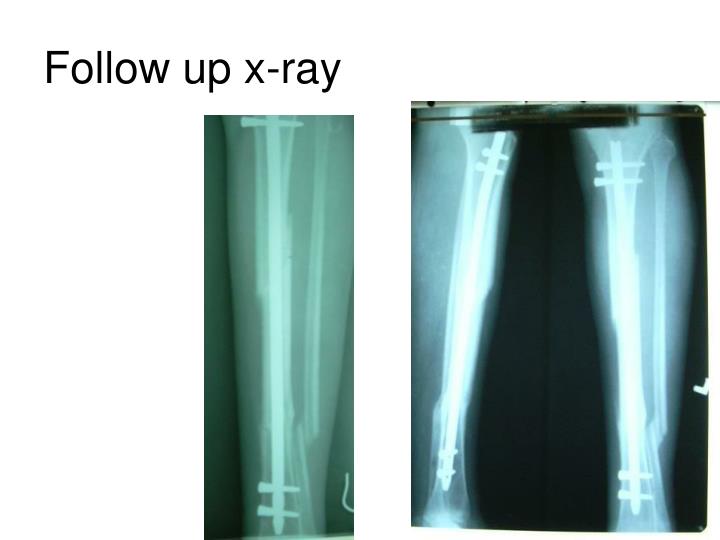This image is a medical slide on a white background, showcasing two x-rays under the title "follow up x-ray" in black font. The x-ray on the left features a single leg bone with the bones clearly visible and a faint silhouette of the surrounding flesh. It prominently shows metallic pins inserted into the bone, with one pin at the top and two pins at the bottom. The x-ray on the right captures both legs, displaying the same visible bones and faint fleshy outlines. In this image, each leg has two pins at the top and two at the bottom, revealing post-surgical fixation. The left x-ray image has a greenish tinge, while the right one has a black background, emphasizing the skeletal structure and the inserted metal pins.